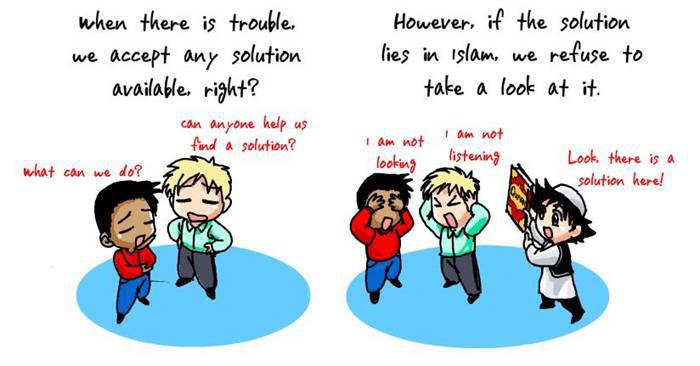The comic drawing, set against a white background, features two main panels. In the left panel, two boys, one in a red shirt and the other in a blue shirt, are standing on a blue circle and conversing. Above them, black text reads: "When there is trouble, we accept any solution available, right?" The boy in the blue shirt asks, "Can anyone help us find a solution?" while the boy in the red shirt responds, "What can we do?" In the right panel, three figures also stand on a blue circle. One character wears a white kurta and a black vest, holding a book (likely the Koran, indicated by a visible "Q"). Above this scene, black text states: "However, if the solution lies in Islam, we refuse to take a look at it." The boy in the blue shirt says, "I am not listening," the boy in the red shirt says, "I am not looking," and the figure in the white kurta asserts, "Look, there is a solution here."